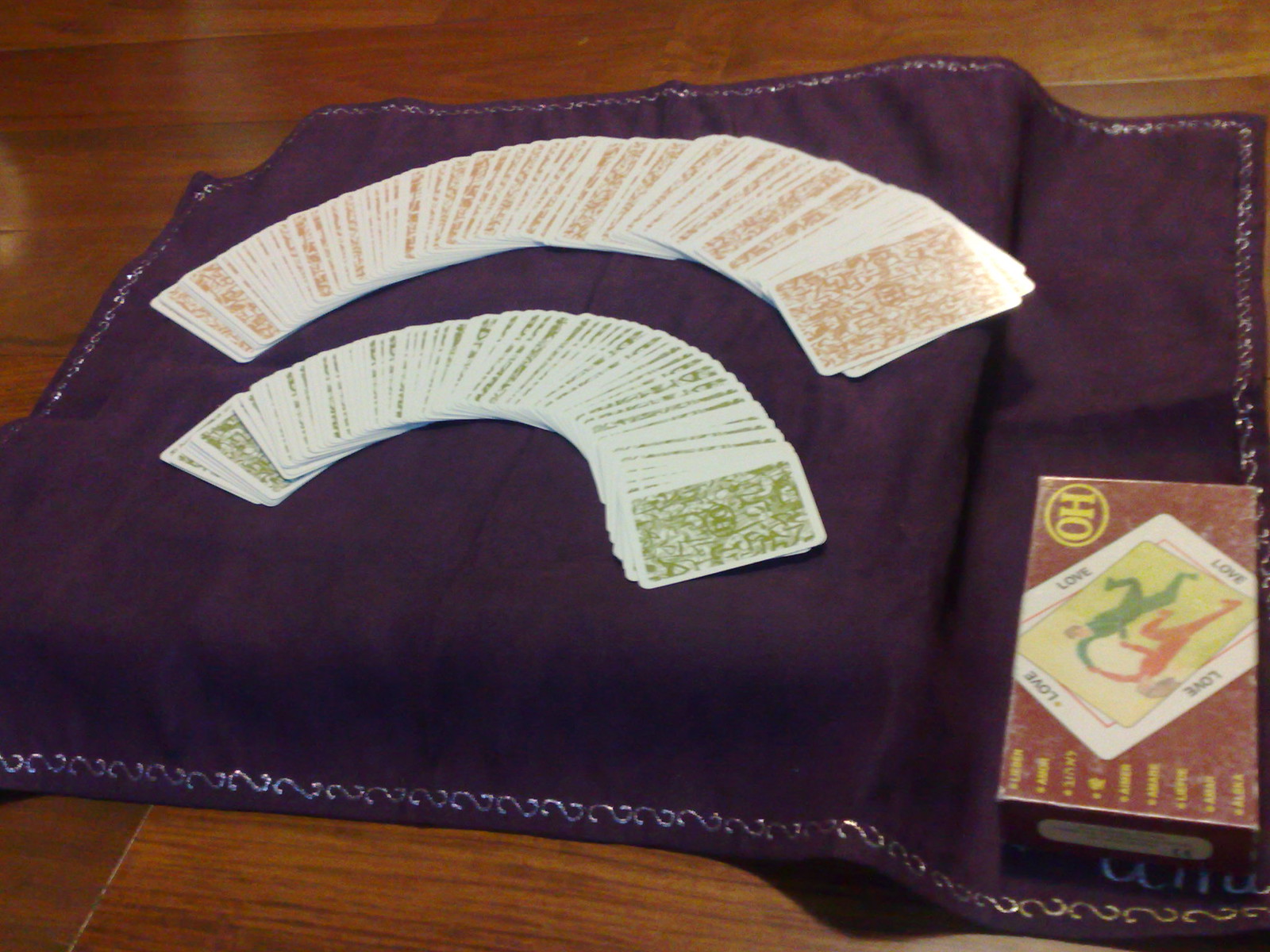The image features two decks of tarot cards arranged on a luxurious piece of dark purple fabric adorned with silver stitching that forms an elegant border composed of numerous 'S' shapes. The cards are meticulously placed in two concentric semi-circles; the outer semicircle is made up of cards with an orangey-brown and white intricate pattern on their backs, while the inner semicircle consists of cards with a similar design in green. Both sets of cards are laid face down, displaying only their ornate back designs. In the bottom right corner, a tarot box is partially visible, with one card showing a charming illustration of two people holding hands and seemingly dancing, identified as the "love" card. Additional writing on the box is indiscernible. The dark purple fabric is elegantly draped over a hardwood table that showcases a light to medium wood tone with darker horizontal grains.